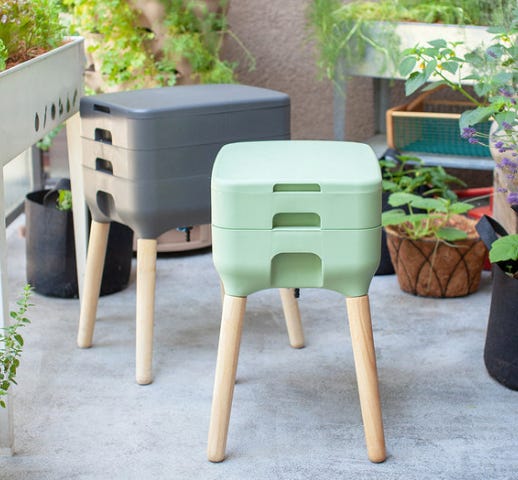This square photograph captures a vibrant outdoor space, likely a back porch or patio, that's been lovingly turned into a plant nursery. The patio, paved with gray stone, is adorned with about 10 to 15 potted plants in various types of containers, including wicker baskets and stylish pots. Ivy and other climbing plants cascade down the walls, enhancing the lush ambiance.

At the center of the patio are two intriguing storage stools. The first stool is pastel green with four white wooden legs and features two compartments—one directly under the handle that lifts to reveal storage space, and another thinner compartment above that. The second stool, a pastel gray, appears similar but includes an additional level, offering four compartments in total. Their design suggests they can be adjusted by adding or removing layers, making them versatile for various gardening tasks, perhaps even storing tools. The meticulously arranged plants and multifunctional stools create a visually appealing and functional gardening space.